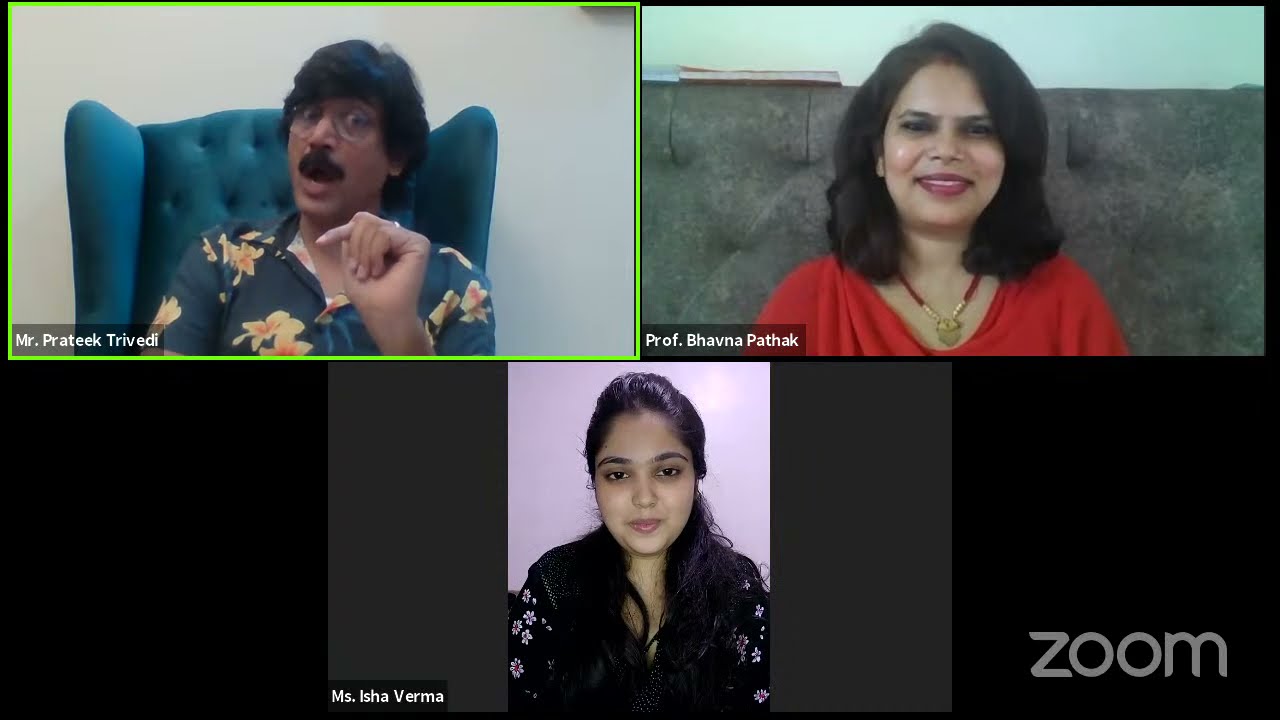This composite image captures a lively Zoom call featuring three individuals of apparent Indian origin. In the upper left frame is Mr. Prateek Trivedi, wearing a blue Hawaiian shirt adorned with yellow flowers, and sitting in a high-backed bluish chair against a white wall. His eyes are wide open behind glasses, and he sports a thick black mustache. Mr. Trivedi's right hand is raised in an expressive gesture, suggesting he is in the midst of a spirited discussion, which appears to amuse the other participants. 

To the right, the top frame shows Professor Bhavana Pathak. She sits on a gray sofa and wears a red blouse paired with a red necklace featuring a gold pendant. Her shoulder-length black hair frames her face as she smiles warmly, displaying high cheekbones and rosy cheeks. 

Centered at the bottom is Ms. Isha Verma, whose long dark hair partially tied, cascades over her shoulders. She wears a black top with floral patterns on the sleeves, looking directly into the camera with dark eyes and an amused expression. The familiar Zoom logo is visible in the lower right corner, reinforcing the context of the image.